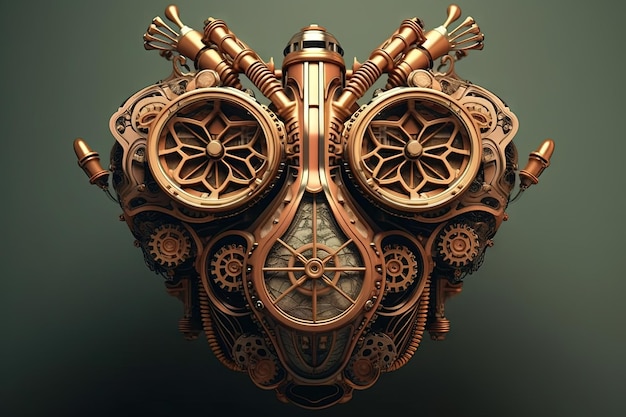The image depicts a detailed, steampunk-inspired object resembling a heart, centered on an olive green background that darkens to nearly black at the bottom. The heart-shaped object, predominantly bronze in color with accents of orange, brushed red, and beige, is intricately assembled from gears, pipes, and various mechanical elements. A dome-like, teardrop-shaped structure sits atop the heart's center, reminiscent of a lightbulb, and extends upwards. Flanking this central structure are smaller, cylindrical objects with trumpet-like ends that protrude on each side, alongside additional lightbulb-like components. Two larger circular forms on either side suggest the left and right ventricles, evoking the anatomical structure of a heart. The complex assembly of gears, hoses, and mechanical parts creates a visually striking piece of steampunk art, set against the richly shaded backdrop.